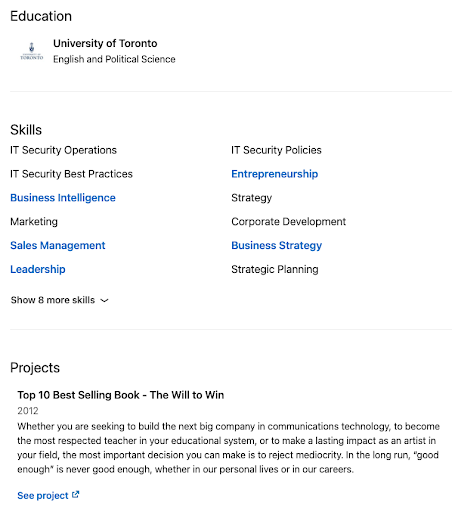The image displays a section of a CV, oriented in portrait format with a plain white background seamlessly blending into the document. 

In the top-left corner, the heading "Education" is prominently displayed. Below this heading, it specifies the "University of Toronto," detailing a focus on "English and Political Science" as the subject of study. A subtle, light gray horizontal line separates this section from the next.

The following section is titled "Skills," encompassing a comprehensive list which includes "IT Security Operations," "IT Best Practices," and "Marketing Strategy." Noteworthy is the differentiation in font color - "Business Intelligence," "Sales Management," "Leadership," "Entrepreneurship," and "Business Strategy" are highlighted in blue, indicating these are areas of particular proficiency for the individual. The remaining skills are: "Project Management," "Financial Analysis," "Strategic Planning," "Customer Relationship Management," "Data Analysis," "Team Building," and "Communication Skills." Additionally, a dropdown option suggests the presence of eight more skills not immediately displayed.

Below this primary skills list, another horizontal gray line serves as a separator, leading into the "Projects" section. This highlights a notable accomplishment: "Top 10 Selling Book, The Will to Win, 2010." Accompanying this title is a brief paragraph providing context about the book. To the right of this paragraph, a blue hyperlink labeled "See Project" with a small upward arrow invites readers to explore further details about the book.